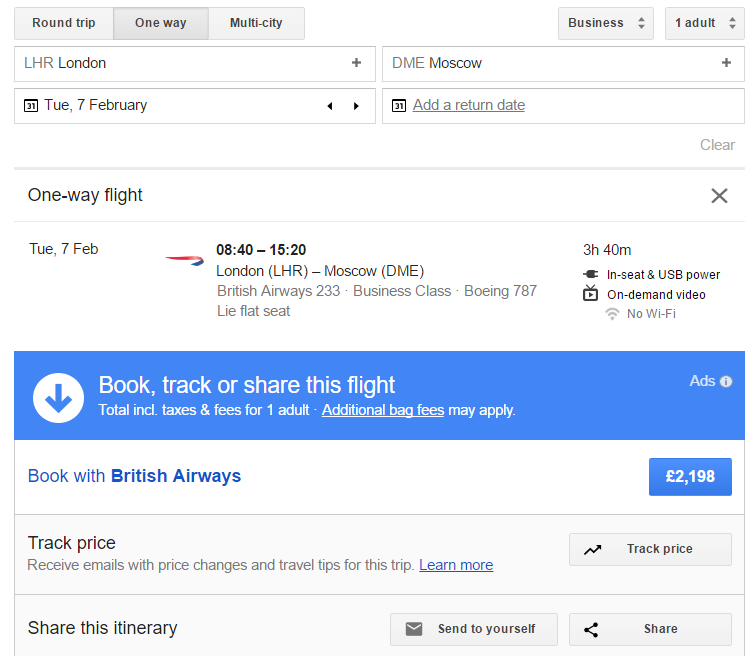This screenshot, taken from a webpage and carefully cropped to exclude browser and web title information, illustrates the process of searching for airline flights. The search parameters, prominently displayed at the top, indicate a one-way journey from London Heathrow Airport to Moscow Airport for one adult, scheduled for February 7th, with no return date selected. 

Below the search section, a flight option is presented: British Airways Flight 233 in business class. This flight departs at 8:40 AM and arrives at 3:20 PM, making for a total flight duration of 3 hours and 40 minutes. Accompanying the flight details is a blue box featuring options to book, track, or share the flight. Booking directly through British Airways will cost £2,198.